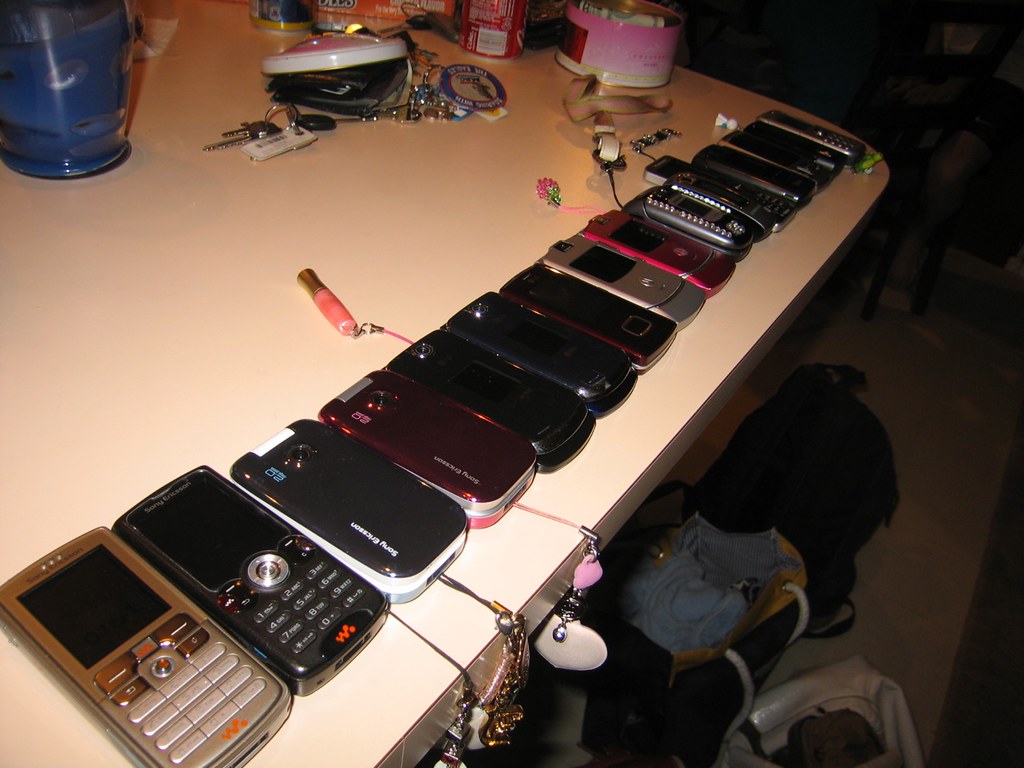The photograph is an overhead, slightly angled view of a cluttered white countertop in a likely dormitory or college girl hangout environment. The countertop is filled with an array of approximately 14 to 15 classic cell phones predominantly from the early 2000s. These include various models such as Sony and Motorola flip phones, many of which have vibrant colors like burgundy, silver, and a standout pinkish red model. The arrangement starts from the bottom left corner and angles up toward the top right, making the phones closest to the camera appear larger. Several phones are adorned with keychain decorations, three of which dangle off the edge of the table. The phones are a mix of classic designs, including some brick phones and bedazzled pieces, all closely packed together. The ivory-colored surface also holds miscellaneous items such as pop cans, keys, a cup, and other bits of metal. Below the table, a bluish floor is visible, scattered with clothes, bags, and other items, enhancing the sense of a lived-in, casual setting.